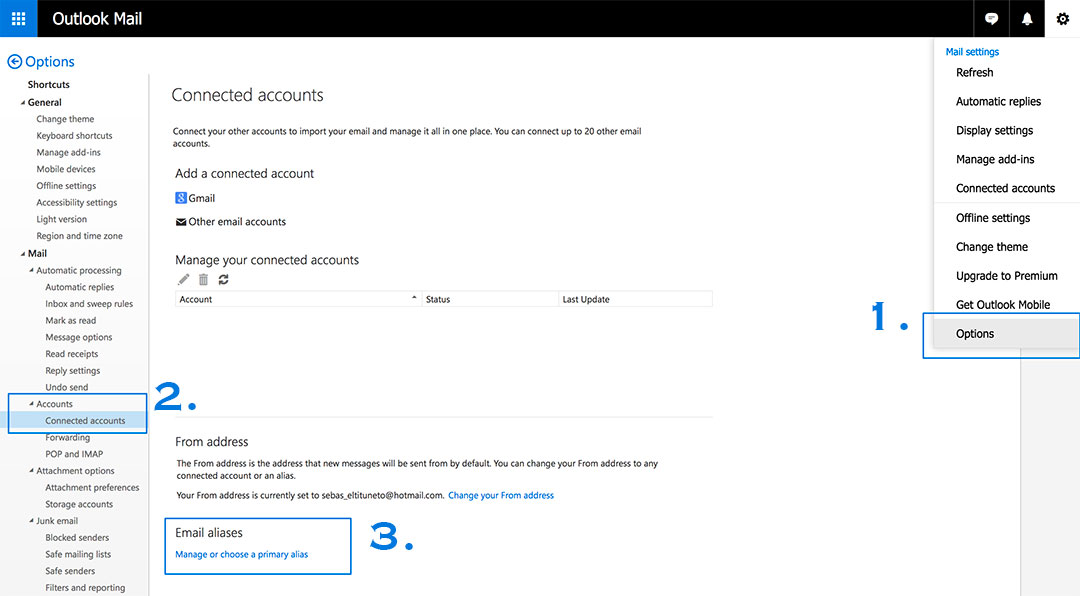The image displays the Accounts, Connected Accounts page within the Outlook Mail interface. On the left sidebar, there is a vertical menu starting with "Options" at the top, followed by "Shortcuts" and "General." Under the "General" category, there are several settings options: Change Theme, Keyboard Shortcuts, Manage Add-ins, Mobile Devices, Offline Settings, Accessibility Settings, Light Version, Region, and Time Zone.

In the main window, the "Accounts" section is prominently highlighted in blue, specifically on the "Connected Accounts" option. The page provides options to "Add a Connected Account," listing Gmail and Other Email Accounts as available choices. Below these options, there is a message indicating "Manage Your Connected Accounts," followed by a statement indicating that no accounts are currently connected.